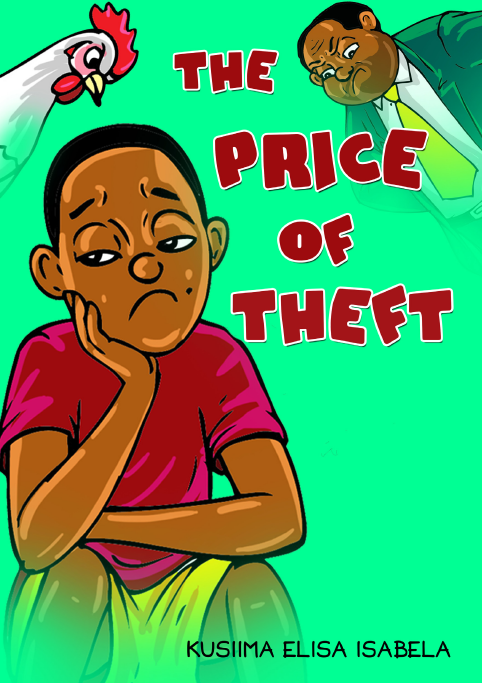The cover of the children's book "The Price of Theft" by Kusima Elissa Isabella features a vivid, cartoon-style illustration. The background is a vibrant green, while the title text is prominently displayed in red with a white outline. In the top left corner, an angry white rooster with a yellow beak and red comb glares downward. Opposite, in the top right corner, an elderly black man in a blue suit, white shirt, and yellow tie also looks angrily towards the center. The focal point of the cover is a melancholic black boy situated in the bottom left, sitting with one hand resting on his face and the other arm crossed over his knees. He wears a pinkish-red shirt and yellow shorts, conveying a sense of regret and sadness. The interplay of green, red, yellow, and other colors creates an engaging and expressive visual narrative.